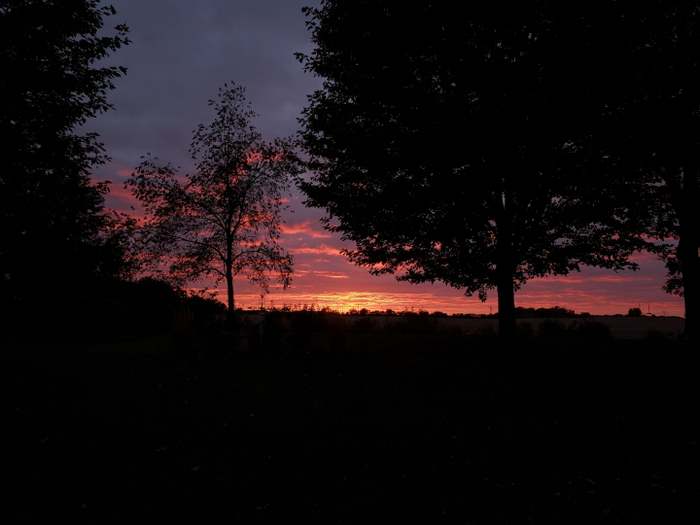This is a vibrant, detailed photograph capturing the breathtaking moment of a sunset transitioning into twilight. The sky is painted with a stunning array of colors: a gradient of gold and orange near the horizon gives way to deep, dark pinks, which then blend into lighter pastel pinks, purples, and finally a grayish-blue hue higher up. The last light of the setting sun casts a bright yellow glow, making its presence distinct even below a layer of clouds. The foreground is dominated by the silhouettes of several trees, their dark forms contrasting sharply against the colorful sky. These trees include a larger, shadowy silhouette, a smaller, straggly tree reminiscent of Charlie Brown’s Christmas tree, and another full-bloom tree. The terrain appears flat with tiny trees dotting the distant horizon. The vibrant colors of the sky and the deep black silhouettes create a striking, lush scene that emphasizes the beauty of nature at dusk.